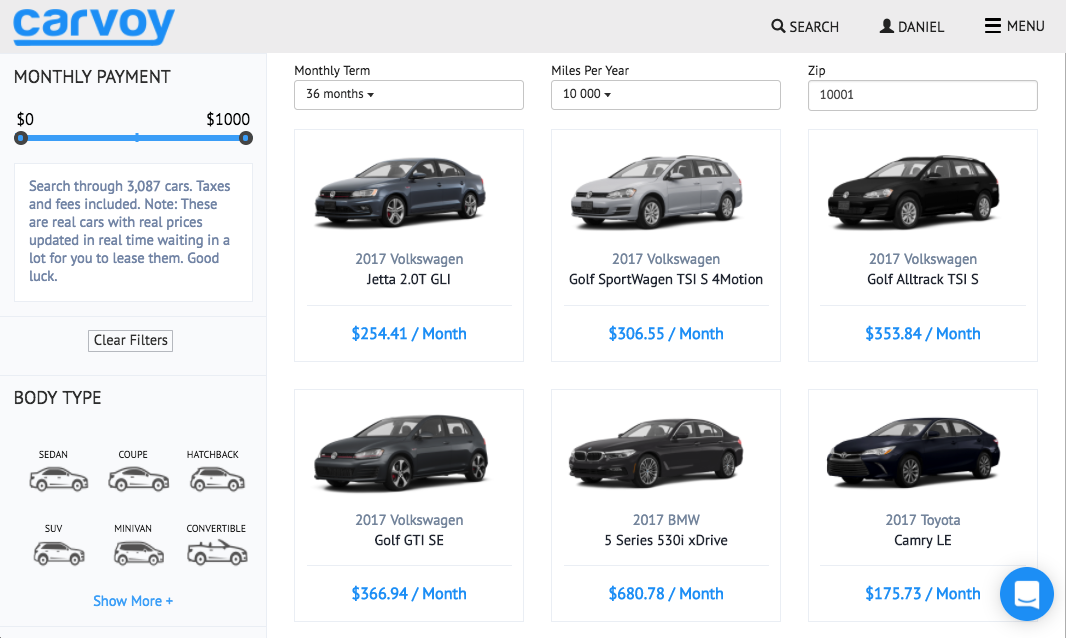The image portrays a user's view of the Carvoy website. At the top, there is a light gray banner featuring blue text on the left side that reads "Carvoy," with the line from the lowercase 'y' extending all the way back to the 'C'. On the right side of the same gray banner, the options "Search," "Daniel," and "Menu" are displayed.

Beneath the banner, a left-aligned section in an even lighter gray background contains black text stating: "Monthly payment from $0 to $1,000, search 3,087 cars, taxes and fees included. Note, these are real cars with real prices, updated real-time, waiting in the lot for you to lease them. Good luck." This section also includes options like "Clear filters" and body types including sedan, coupe, hatchback, SUV, minivan, and comfortable, with a "Show more" link in blue text accompanied by a plus sign.

The main part of the page has a white background. It features drop-down menus for "Monthly term: 36 months," "Miles per year: 10,000," and a zip code field set to "10001." Displayed are two rows of car listings. The top row includes: 
1. 2017 Volkswagen Jetta
2. 2017 Volkswagen Golf SportWagen
3. 2017 Volkswagen Golf Alltrack

The bottom row presents:
1. 2017 Volkswagen Golf GTI SE
2. 2017 BMW 5 Series 530i xDrive
3. 2017 Toyota Camry LE